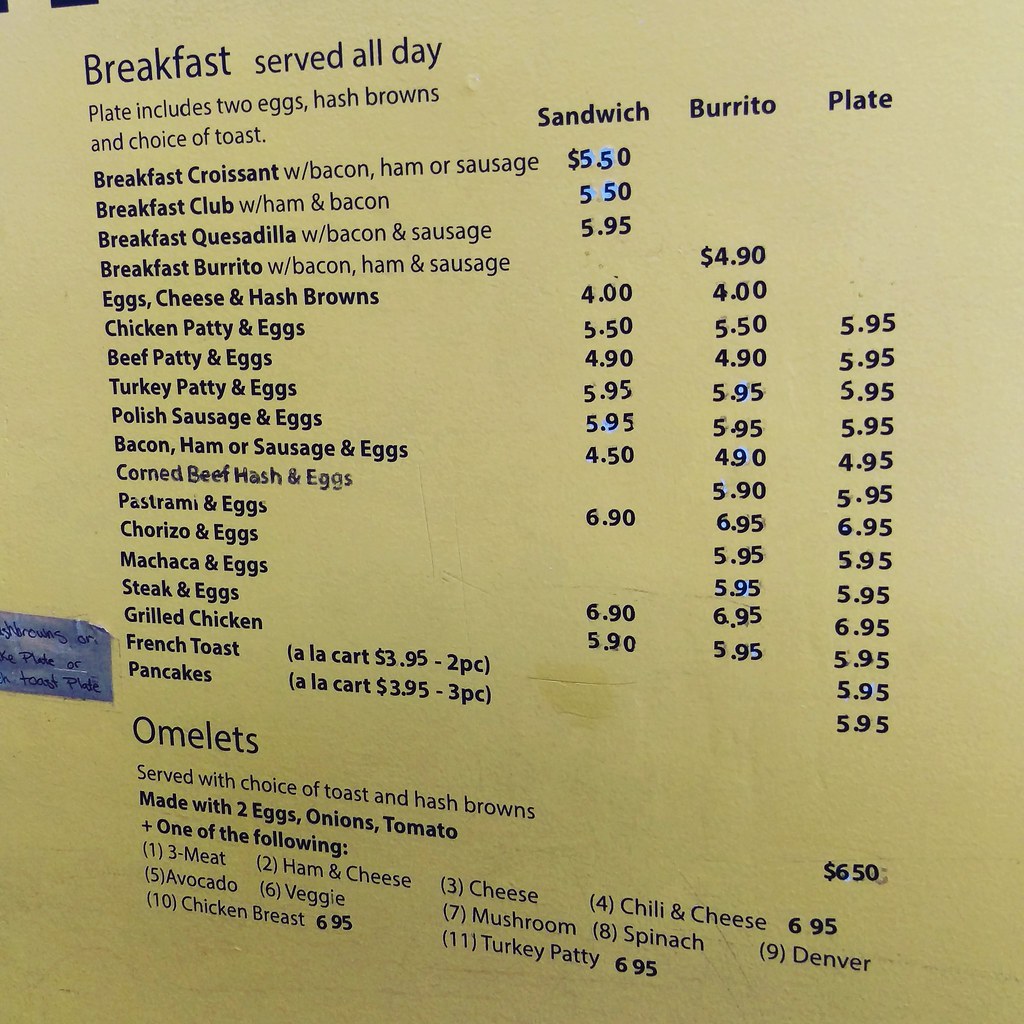This image showcases a detailed breakfast menu set against a light yellow background. The menu items are listed systematically on the left. Adjacent to these items are three distinct columns of pricing details. The first column provides prices for items prepared as sandwiches, the second column lists prices for the same items offered as burritos, and the final column includes prices for complete plated meals.

The menu features a diverse array of breakfast options, ranging from croissants to breakfast quesadillas, including choices like bacon, ham, eggs, and corned beef. There is a special section for omelets, priced at $6.50 each. These omelets come prepared with two eggs, onions, tomatoes, and a choice of one additional ingredient from a variety of options such as ham and cheese, mushrooms, or chili and cheese. Each omelet is served with a choice of toast and hash browns, offering customers a hearty and customizable breakfast option.